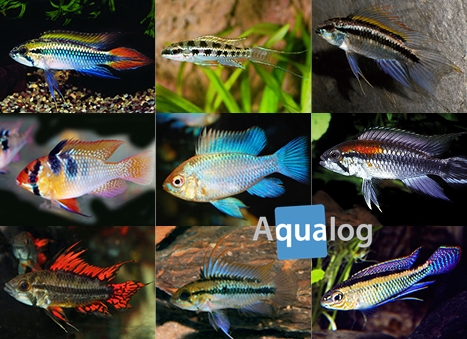This image is divided into nine separate squares, each showcasing a distinct South American Dwarf Chinchillid fish, likely small in size, akin to minnows or goldfish. In the top-left square, a silver fish with a prominent black stripe down its center is displayed, featuring yellow on its top fin and red on its tail fin. Adjacent to this, the second square shows a black and silver fish adorned with black splotches amidst green aquatic plants, and a long, flowing tail fin. The third fish on the top row is silver with two black lines on its side and one across its top fin.

Proceeding to the second row, the first image reveals a vivid red, black, and yellow fish with a tail that's a silverish yellow shade. The middle square presents a uniformly silverish-blue fish. The final fish on this row is silver with a central black stripe, a black marking on the base of its top fin, and a red patch.

On the bottom row, the first fish is a dark silver with black splotches, displaying a striking solid black line down the center and bright red and black fins. The middle square shows a silver fish with a large solid black line down the center and a blue top fin. Its top fin has a black line crossing it. The final fish in the bottom-right is silver, marked by a black stripe along its top and dark blue, almost purple fins.

In the sixth, seventh, and eighth squares, the name "AQUALOG" appears in white text against a blue background.